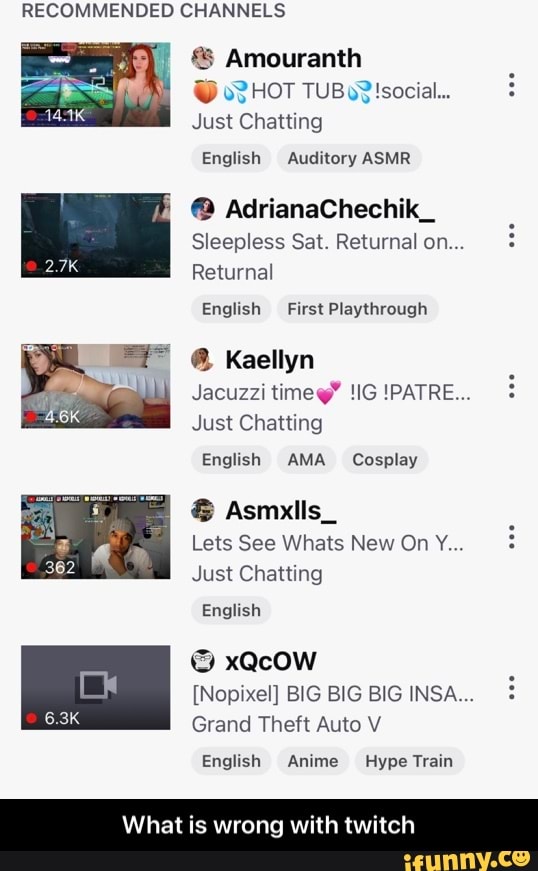This is a detailed screenshot of the Twitch app's interface, showcasing various recommended channels at the top of the screen. There are five distinct thumbnail images, each representing a different stream. 

1. The first thumbnail features a red-headed woman wearing a green bikini, set against a colorful background that suggests she is playing a game. The stream has 14.1K viewers as indicated by a red dot and is hosted by "Amaranth," categorized under "Hot Tub," "Social," "Just Chatting," with options to switch to English and "Auditory ASMR."

2. The second thumbnail appears to display gameplay footage with the title "Adriana Chechik Sleepless Saturday." The stream is focused on the game "Returnal," marked as an English "First Playthrough."

3. The third thumbnail depicts a woman in bra and underwear lying on a couch. The stream is titled "Kaylin Jacuzzi Time" and falls under the "Just Chatting" category.

4. The fourth thumbnail shows two men side by side, accompanied by the stream title "Let's See What's New On." This stream is also categorized as "Just Chatting" with an option for English.

5. The fifth thumbnail features an image of a video camera with the title "Big Big Big Insta." The stream is labeled under "Grand Theft Auto V."

At the bottom of the screenshot, there is a caption questioning the content on Twitch, stating, "What is wrong with Twitch?"